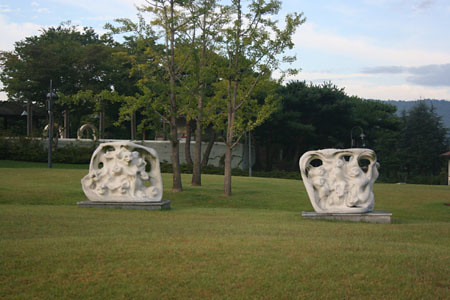The photograph captures a dimly lit scene, likely taken near sunset, in what appears to be a park or expansive field edged by dense forest-like trees. The background features large conifer trees, contributing to the darker, shadowed atmosphere with hints of orange from the setting sun. In the foreground, two mysterious white sculptures sit atop stone platforms on uneven, grassy terrain reminiscent of small rolling hills. The sculptures, described as having a white or creamy hue, appear to be inverted versions of each other, with possible face-like features and a distinct, spiked texture. To the left and right, there are additional details including a white fence or wall, light posts, and a few hoops, adding to the intricate setting of this intriguing outdoor space.